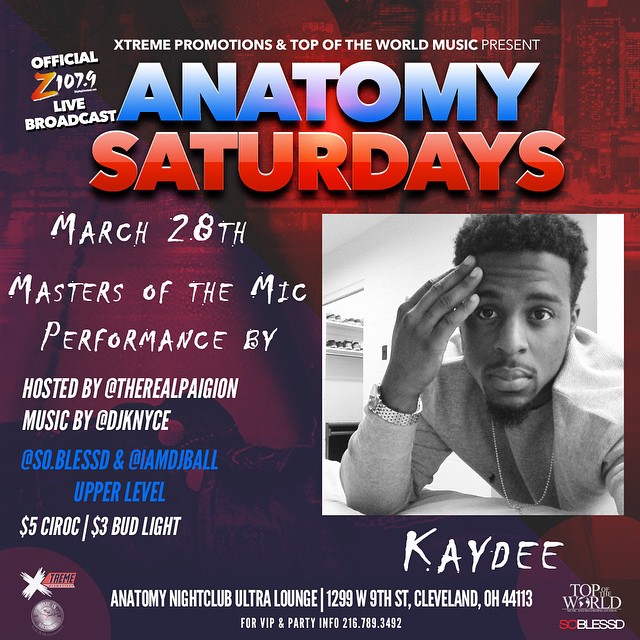This image is a detailed advertisement for an upcoming event titled "Anatomy Saturdays" taking place on March 28th at the Anatomy Nightclub Ultra Lounge in Cleveland, Ohio. At the very top, the text reads "Extreme Promotions and Top of the World Music Present" in bold, all-capital letters. The event name "Anatomy Saturdays" is prominently displayed in a bold, 3D graphic font, with "Anatomy" written in blue and "Saturdays" in red.

The central portion of the poster features a striking black-and-white close-up photograph of an African-American man, identified as KD (spelled "K-A-Y-D-E-E" in some graphic art). The man has short black hair, a short beard with a mustache, and is seen wearing a gray sweatshirt, a chain, and a gold watch on his right wrist. He is leaning forward, with his right hand touching his forehead.

Below the event title, more details are provided in white text, stating "March 28th - Masters of the Mic Performance." The event is hosted by The Real Paigion, with music by DJ Nice (spelled "K-N-Y-C-E"). There are further mentions of social media handles "@SoBlessed" and "@IAmDJBall Upper Level" in blue text. The bottom of the poster lists $5.00 Ciroc and $3.00 Bud Light specials.

The background of the poster features a mix of red, purple, and blue hues, creating a vibrant and eye-catching design. Additional information, such as the official Z107.9 Live Broadcast and various promotional logos, is included towards the bottom. The address of Anatomy Nightclub Ultra Lounge is also provided, making it clear where the exciting event will take place.